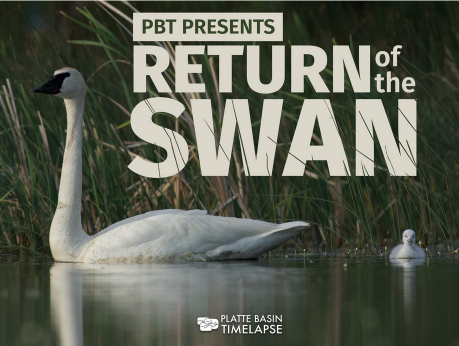The image appears to be an advertisement for a TV show. It is vertically oriented and showcases a serene nature scene. In the foreground, a white adult swan with a long neck and a black beak floats gracefully on dark green water. Slightly behind it is a smaller, baby swan with a tinier, red beak. Both birds are reflected beautifully in the water beneath them. The background is filled with tall, thin blades of vibrant green grass. Overlaying the scene is the text: "PBT presents Return of the Swan" at the top of the image, with "Return of the Swan" in a thick white font, and "PBT presents" in green with a white border. At the bottom, it reads "Platte Basin Time-lapse," completing the promotional message.